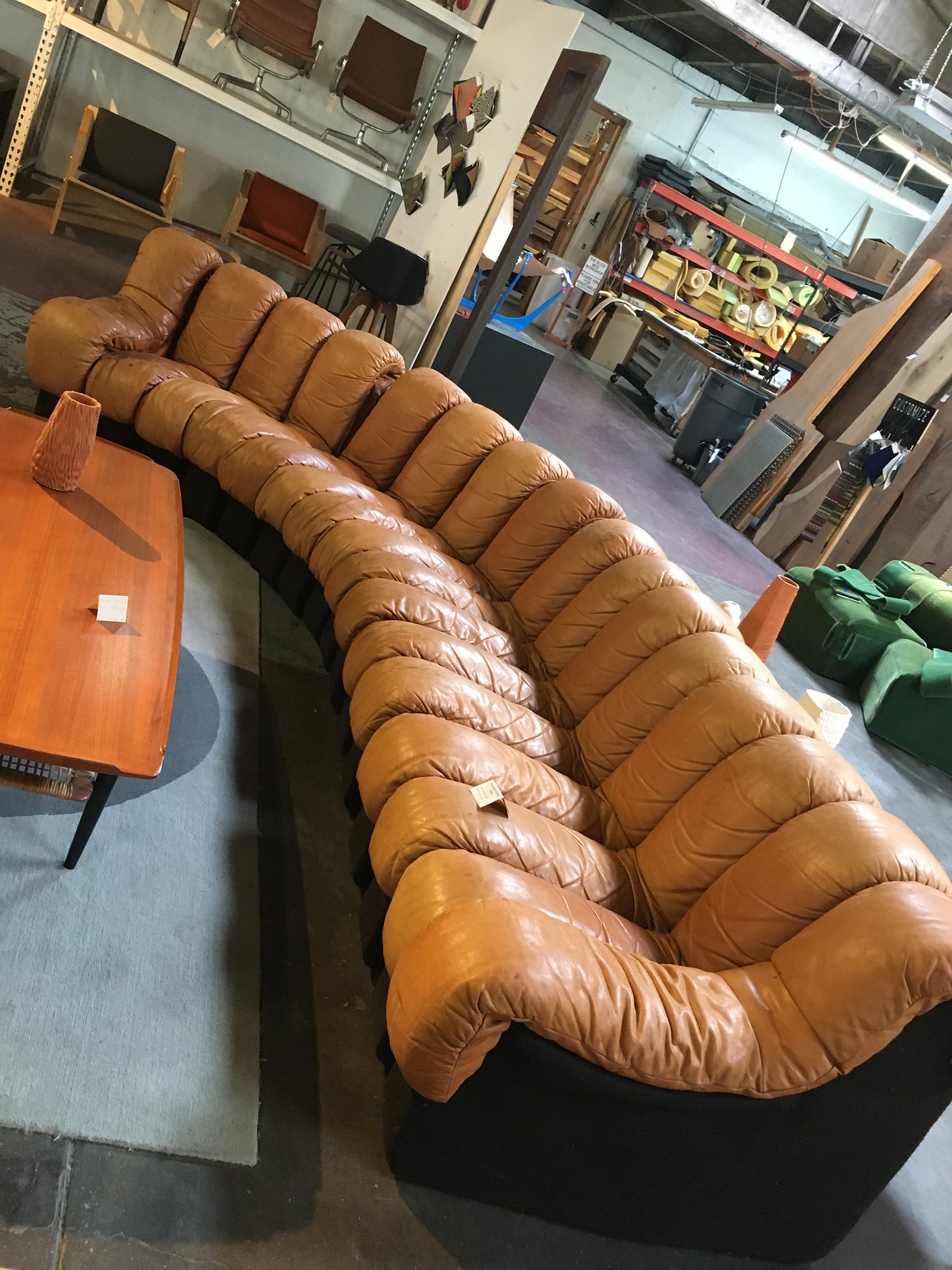The image, taken inside a slightly askew furniture store or warehouse, reveals a detailed scene centered around a very long, curved sectional sofa featuring orange or tan leather with clearly defined individual seating divisions and a dark brown base. The sofa stretches from the foreground on the right to the back left of the photo. Situated in front of the sofa on a blue-gray area rug is a wooden coffee table with a medium brown top and brown metal legs, under which sits a basket. The table is adorned with a brownish-orange vase and a folded white paper. In the background, a wall lined with shelving displays a variety of chairs, including swivel chairs with metal arms and fixed chairs with wooden arms. To the back right, another room filled with foam and packing materials signals a warehouse-like area for workers. Scattered throughout the store are additional pieces of furniture, including green upholstered chairs.